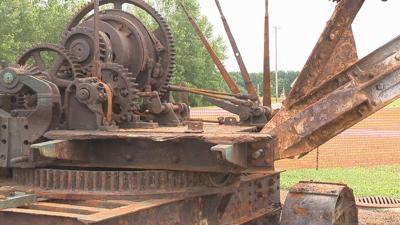The photo showcases a rusted, antique piece of mechanical equipment, possibly farm machinery, set in a rustic outdoor environment. Its dark brown and gray metal structure is heavily speckled with rust, giving it an aged and weathered appearance. Prominent features include several intricate gears lined up side by side, sharp-edged components, and long spiky elements interspersed among the wheels and thick metal pipes. The machinery appears to date back many years and could have served agricultural purposes, such as planting or soil preparation. In the background, lush green trees frame the scene, which includes a hazel-white overcast sky, a dirt road, and distant elements like a light pole and netting. The right side of the image is particularly bright, likely due to sunlight reflecting off the machinery, and hints of a track field or cultivated plots can be seen nearby.